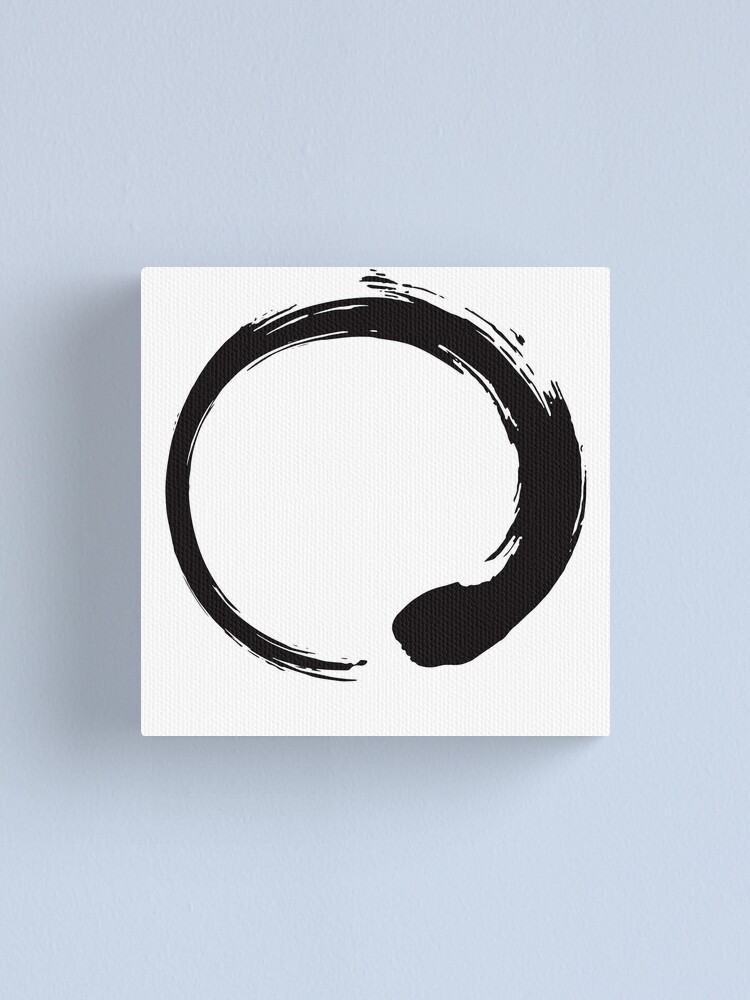The vertically aligned rectangular image features a solid medium gray background, likely intended to resemble a wall. Centered on this gray backdrop is a bright white, square canvas print that adds a stark contrast to the wall. The canvas hosts a single, dynamic black paint stroke that forms an almost complete circle, with a noticeable gap at the bottom. This circular stroke exhibits distinct variations in its thickness: it starts thick on the lower right, remains robust as it arches upward and leftward, and then gradually thins out as it descends the left side. The paint stroke, which appears textured, gives the impression of being executed in one continuous motion, showcasing visible brush strokes along its edges. A subtle drop shadow is evident on the left and bottom edges of the canvas, enhancing the sense of depth and dimensionality.